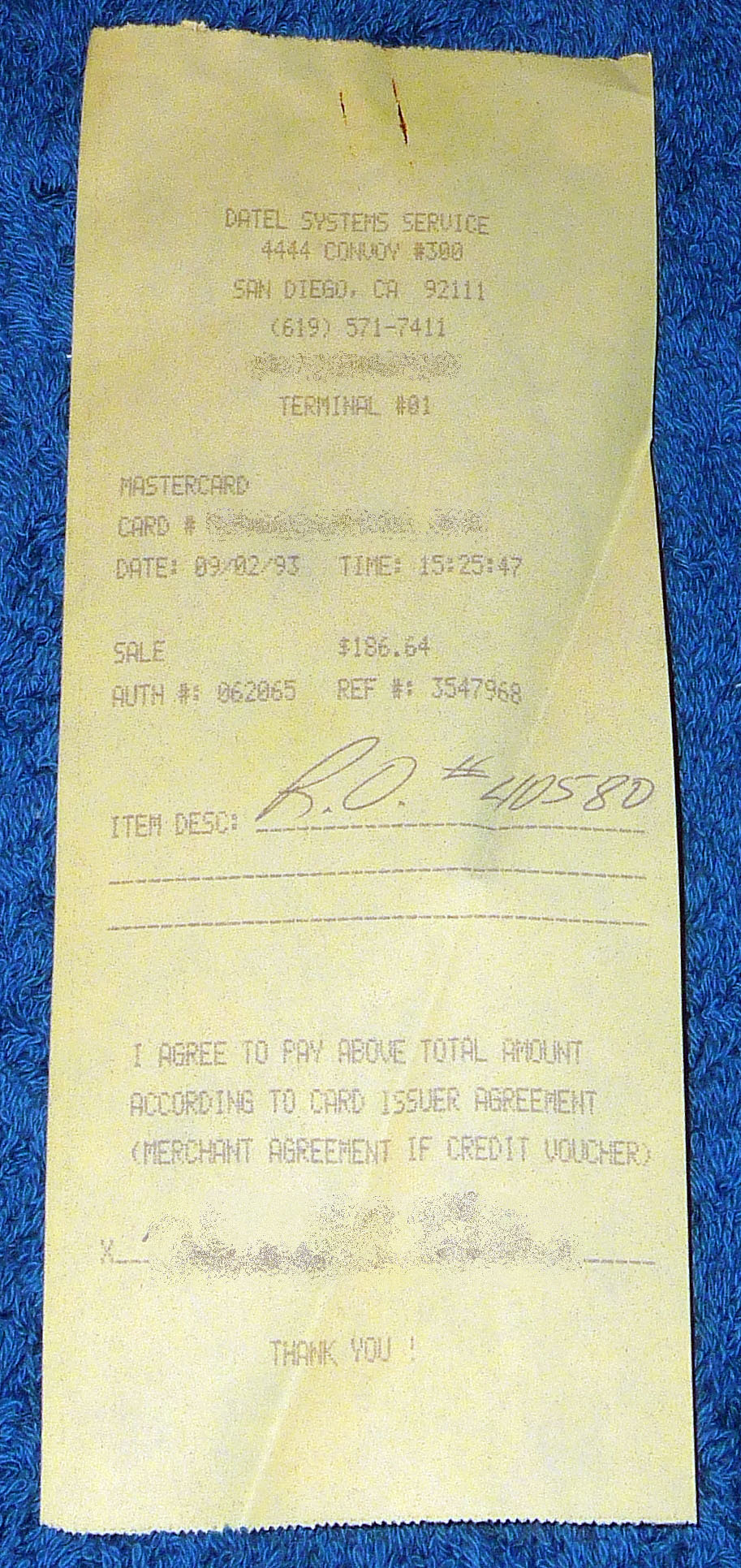This image showcases a detailed view of a receipt from Daytel Systems Service located in San Diego, California, dated September 2, 1993. The receipt, printed on standard white receipt paper, is positioned on a bright royal blue and black speckled Formica table. Evident from a pronounced diagonal crease, the receipt appears to have been folded and then unfolded. The customer settled their bill of $186.64 using a MasterCard, with the card number artfully obscured for privacy. Notably handwritten in pen, the line item reads "R.O.40580." While the bottom of the receipt includes a space for the customer's signature, the signature itself is heavily blurred, likely due to exposure to moisture, making it largely illegible.